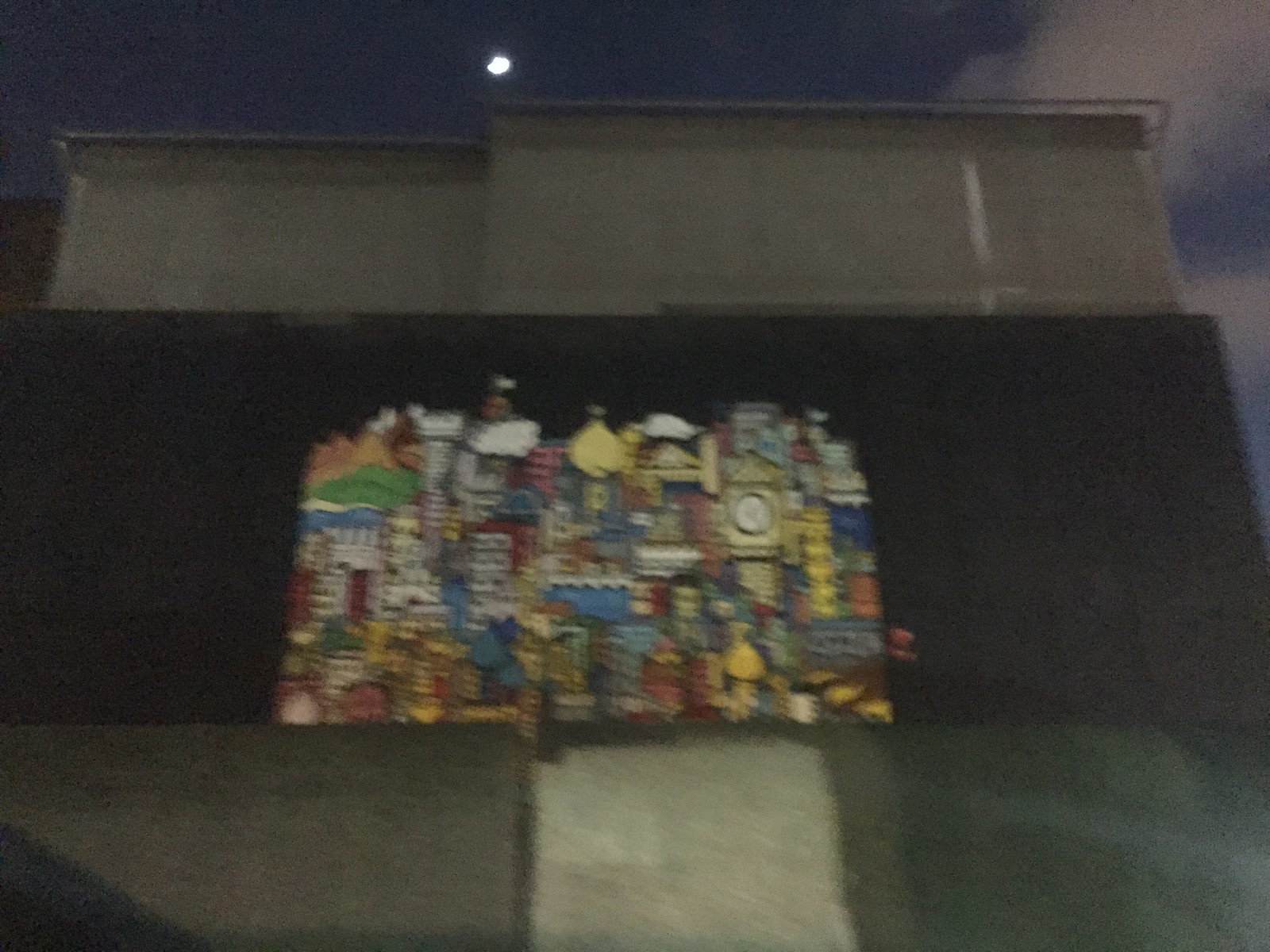This photograph captures a mural on the side of a building during nighttime, with the moon faintly visible at the top, adding a serene light to the scene. Although the image is blurry and the details of the mural are hard to discern, the mural is notable for being sizable yet not covering the entire wall. The mural is set against a background of a black horizontal line that wraps around the building. Nearby, two adjacent structures with a distinct square shape, likely apartments, form part of the setting, with one building appearing slightly separated from the other. This creates a backdrop that frames the mural and contextualizes the urban environment in which it resides.